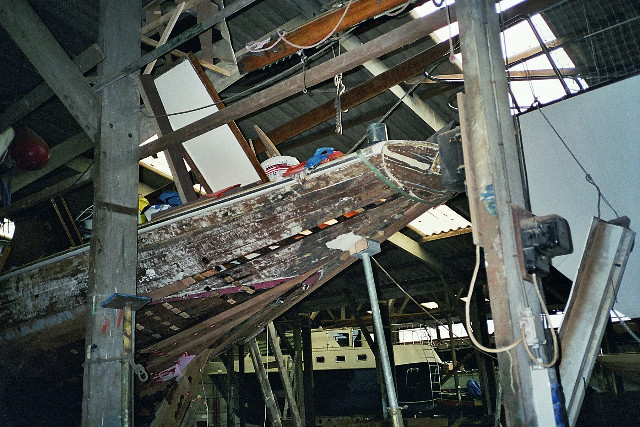The image depicts a scene within a large, partially open indoor area that seems to blend features of both an industrial site and an old seaport dock. At the forefront, there is a section of wooden bleachers or elevated walkways, many of which have decayed and collapsed over time. These wooden structures are supported by both concrete and wooden poles that resemble light poles, suggesting an ongoing or abandoned renovation effort. The area includes an electrical outlet covered with a meter further adding to the sense of disrepair. 

Scattered around the central area are several buckets, adding to the cluttered and neglected atmosphere. The background reveals the interior section with a roof showing visible decay, including an opening, and structural elements like exposed wooden planks and wires. There is also red, white, and blue paint seen on different wooden parts.

Prominently in the distance stands a white and blue boat, identifiable by the ladder placed at its stern. This boat appears to be undergoing refurbishment, evidenced by the surrounding equipment. The environment suggests a blend of industrial decay and a touch of maritime activity, hinting at a potential seaport dock area that has seen better days.